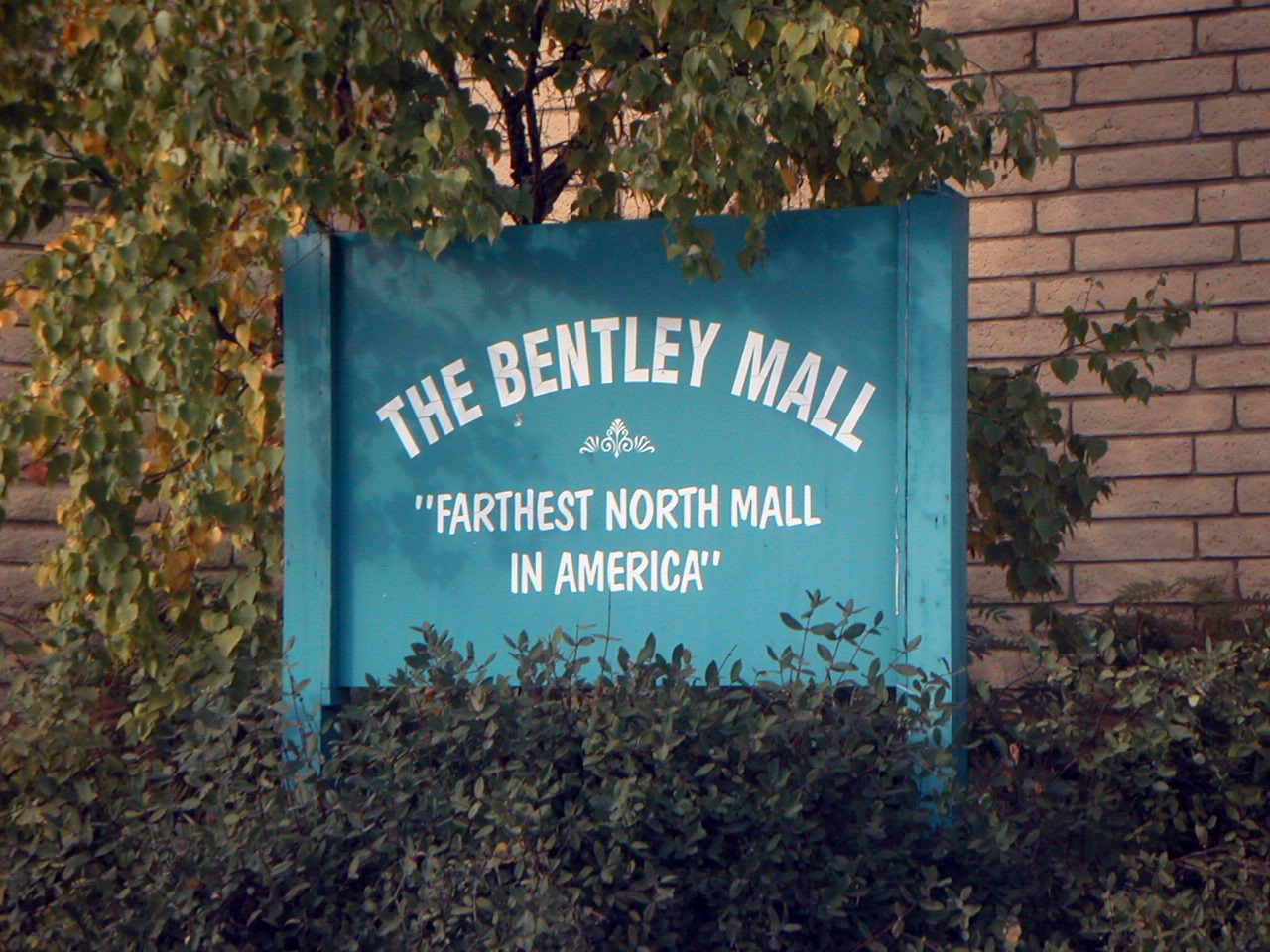This is a color photograph capturing a blue wooden sign positioned in front of a light brown brick building. The bricks are notably longer and lighter in hue than typical bricks. The sign, painted in a robin's egg blue color, stands prominently amid some green bushes, with a small tree—possibly a dogwood—flanking it from behind. The sign, supported by two wide wooden posts, features white lettering in all capital letters that arch across the top reading "THE BENTLEY MALL." Below the main text, there's a small fleur-de-lis design, followed by the phrase "FARTHEST NORTH MALL IN AMERICA" in slightly cartoony white letters enclosed in quotation marks. The tree behind the sign, with its green and brownish-yellow leaves, rises to a height of about 10 to 12 feet and has a thin, narrow trunk. This picturesque scene, situated in front of the light brown brick wall, evokes a sense of northern charm and tranquility.